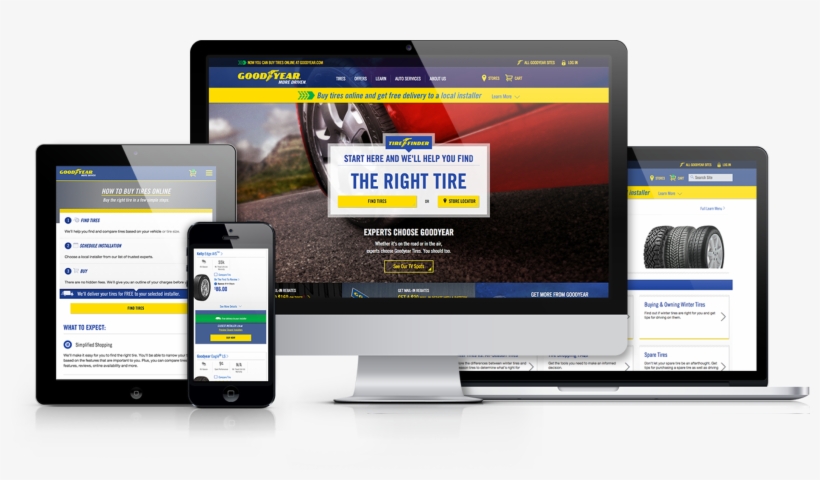Here's a detailed and cleaned-up caption for the image:

---

This image showcases an online advertisement for Goodyear tires, prominently displayed across multiple digital devices. Centrally featured is a computer monitor displaying the Goodyear logo in vibrant yellow in the upper left corner. The screen highlights a striking image of the rear of a red car, with a significant focus on the tire. The central text reads "Find the right tire" with an encouragement to "Start here, and we'll help you find the right tire." Below, clickable buttons for "Find Tires" and "Store Locator" are prominently placed, followed by the slogan "Experts choose Goodyear."

To the left of the monitor sits a black iPad, featuring detailed information on various tire options and navigation links to assist users in finding suitable tires. Adjacent to the iPad, partially overlapping it, is a black smartphone displaying a close-up of a tire along with its price, emphasizing Goodyear's online shopping experience.

Behind the central computer monitor, an open laptop’s screen is visible. The laptop has a black top bezel and a silver bottom casing. On this screen, you can see three tires aligned in a row accompanied by information regarding winter and spare tires, reinforcing Goodyear’s diverse tire offerings.

Each device effectively illustrates Goodyear’s digital presence and user-friendly interfaces aimed at helping customers find and purchase the perfect tires for their needs.